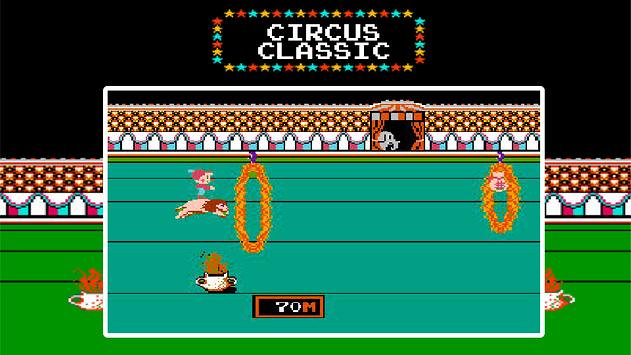The image depicts a nostalgic scene from an old computer game titled "Circus Classic," displayed prominently in white text with a border of multicolored stars—yellow, red, and blue—set against a black background. The primary focus is a 2D screen featuring a circus performance. In this screen, a lion, carrying a small boy or clown, is seen leaping through a flaming hoop on the left, with another flaming hoop visible to the right. The bottom of the screen displays "70M," where the 70 is in white and the M in red, indicating some form of progress or distance within the game. The circus arena has a bright green backdrop, with indistinct figures representing the audience. An additional layer in the image shows another similar scene, reinforcing the classic gaming style and primitive graphics reminiscent of early computer games.